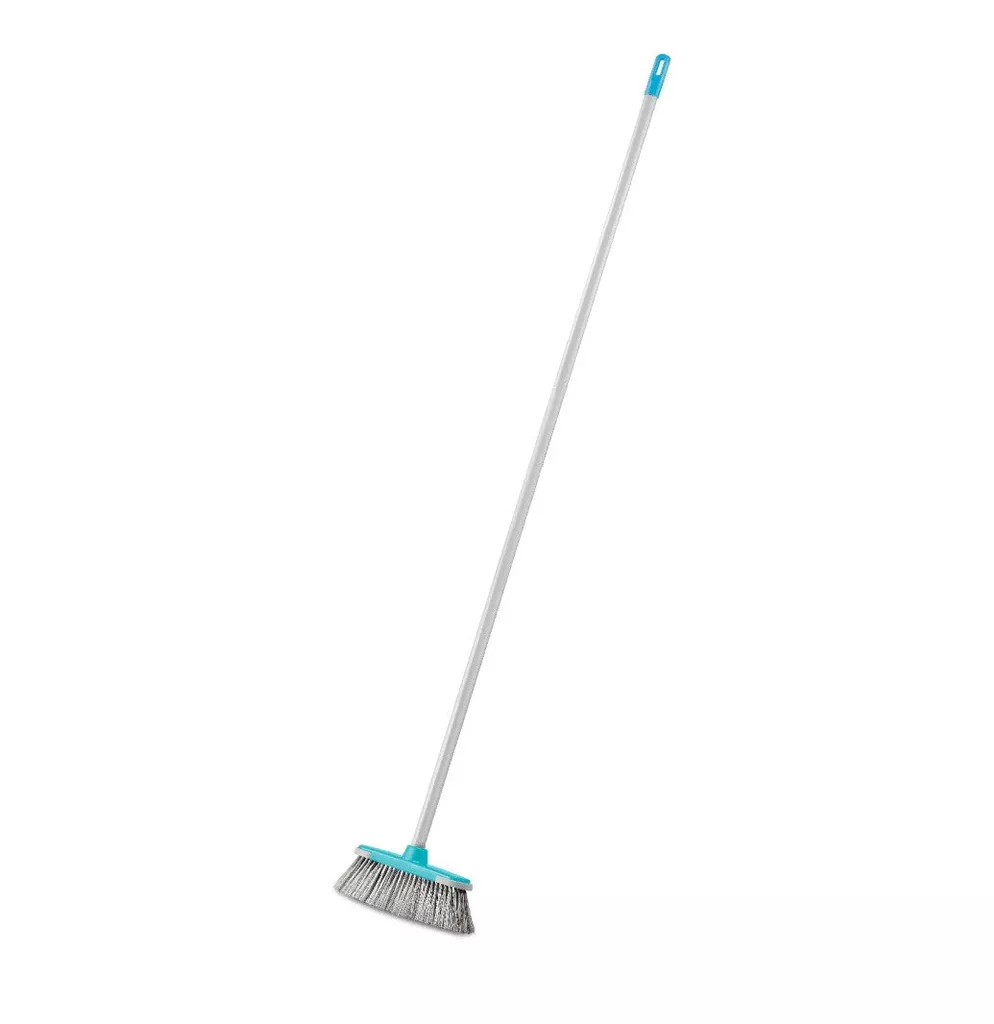The image depicts a simplistic yet oddly proportioned broom on a plain white background, giving it a product promotional feel. The broom is oriented diagonally, extending from the lower left to the upper right, and features an unusually long and thin handle, which is light silver-gray in color. At the top, the handle ends with a turquoise blue plastic tip that has a rectangular hole for hanging. The lower end of the handle is attached to a narrow, flat plastic edge in the same turquoise shade, from which bristles extend. The bristles are light gray and appear somewhat fuzzy, as though they already contain dust. The broom’s bristles are short and compact compared to its overall length, and the entire broom is shown at an angle, adding to its exaggerated dimensions. This makes the broom appear taller than a person, comically amplifying its size in relation to the standard utility tool.